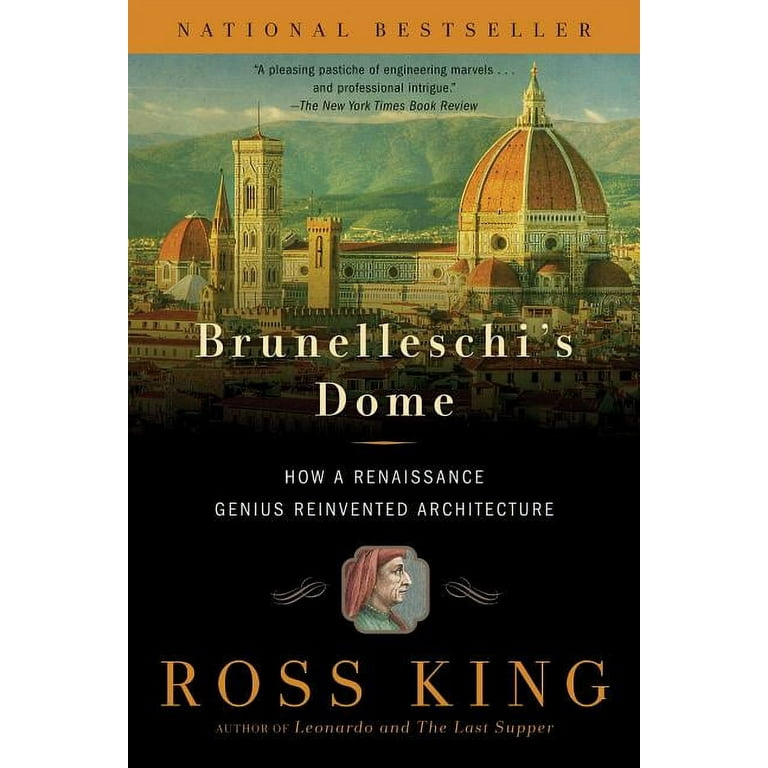The book cover showcases a vibrant and detailed image that commands attention. At the very top, there's a gold and brown bar featuring the text "National Bestseller" in bold black letters. Directly beneath this bar, a review from The New York Times Book Review states, "A pleasing pastiche of engineering marvels and professional intrigue," also in black text.

The central part of the image reveals a picturesque scene of a historic village. Dominating the village is a large, intricate cathedral with a prominent dome and towers. Surrounding the cathedral, smaller tan buildings with orange rooftops add to the charm of the scene. In the background, a sprawling green mountainside, lush with vegetation, ascends towards a blue sky dotted with white clouds.

The book's title, "Brunelleschi's Dome," is prominently displayed in white text across the middle of the image. Below the title, the subtitle, "How a Renaissance Genius Reinvented Architecture," is written in smaller white letters. Towards the bottom of the cover, against a black backdrop, is the image of a man in profile, adorned with a red headdress and wearing a green collared shirt. Flanking the man's image are two white designs, which resemble stylized plus signs with intricate details.

At the very bottom, the author’s name, "Ross King," is written in a striking gold text. Beneath his name, it notes that he is the author of "Leonardo and the Last Supper," also in gold text.